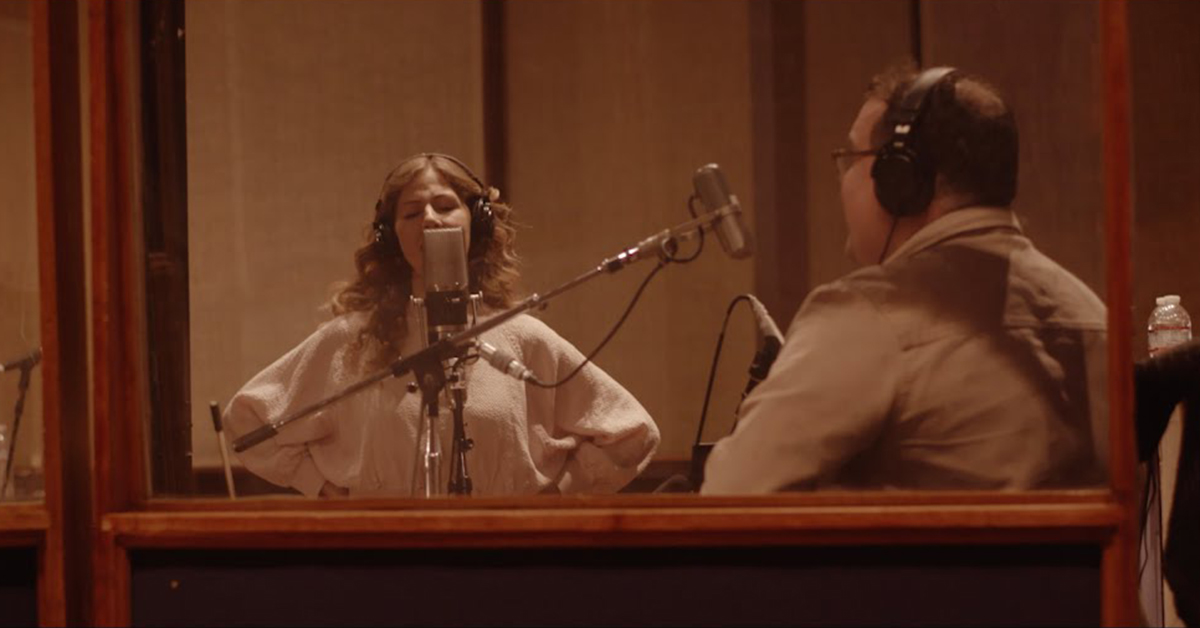In the photograph, two individuals are captured inside a recording booth framed by a wooden panel with a dark black bottom and a transparent glass or acrylic upper section. The panel partially obscures the booth, allowing a glimpse of the man's back from the right side. The man, positioned towards the back right corner, has brown hair, wears glasses, and sports black over-the-ear headphones. Dressed in a long-sleeve white button-down shirt, he sits in front of a microphone on a stand. To his left, a woman with long, light brown or reddish hair, also wears black headphones and a white, flowy linen top. With her hands on her hips and her eyes closed, she appears to be singing into a more sophisticated microphone. The image conveys the dynamic activity within the recording studio, with both individuals engaged in their respective audio tasks.